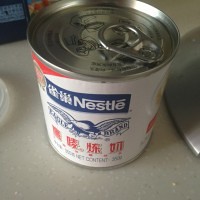The image is a small, square-framed photograph featuring a lightly colored, gray to off-white countertop as its background. The primary subject of the image is a short tin can, positioned at a slight downward angle, giving a clear view of its top and front. The top of the can is intact with its flip lid still sealed. The front label of the can is predominantly white, accented with a blue banner. While most of the text on the label is blurred and unreadable, the blue banner prominently displays the word "Nestle" in the company's distinctive font.